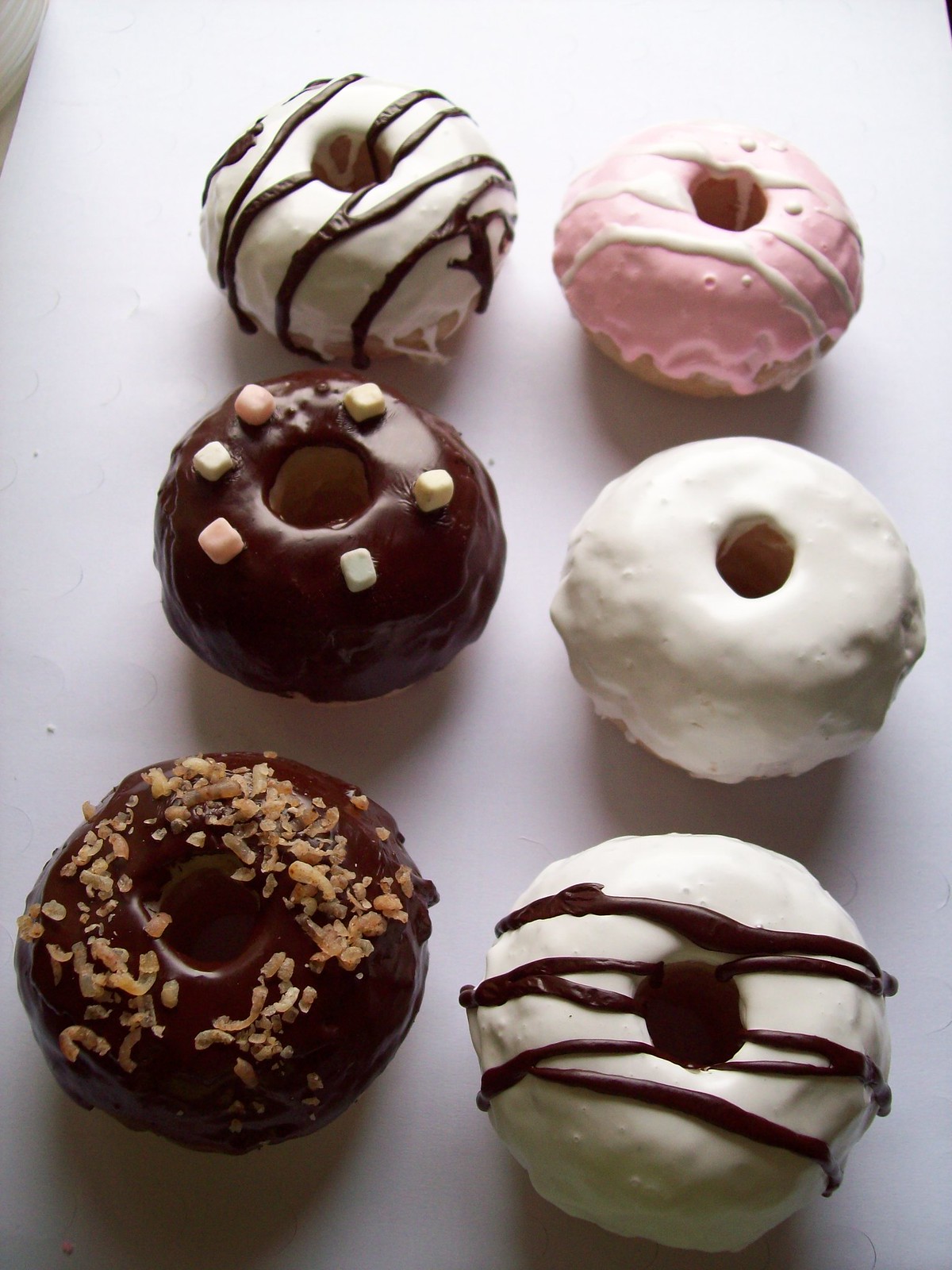The photograph captures six elegantly frosted doughnuts arranged in two columns on a white surface, giving the image a bright and clean aesthetic. Starting from the top of the left-hand column, the first doughnut is adorned with white frosting and drizzled with chocolate stripes. Below it, the second doughnut features rich chocolate frosting topped with six cube-like marshmallows. The third doughnut in this column boasts chocolate frosting sprinkled with what appears to be toasted coconut or shredded nuts.

In the right-hand column, the top doughnut is covered in pink icing, likely strawberry, with white stripes drizzled over it. The middle doughnut in this column is simply dipped in white frosting, giving it a sleek and minimalistic look. The bottom doughnut mirrors the first in the left column, with white frosting decorated with chocolate drizzles. The image is slightly angled, showing part of the tabletop and a couple of tiny crumbs or frosting splashes on the left-hand side, enhancing the casual yet appetizing presentation.